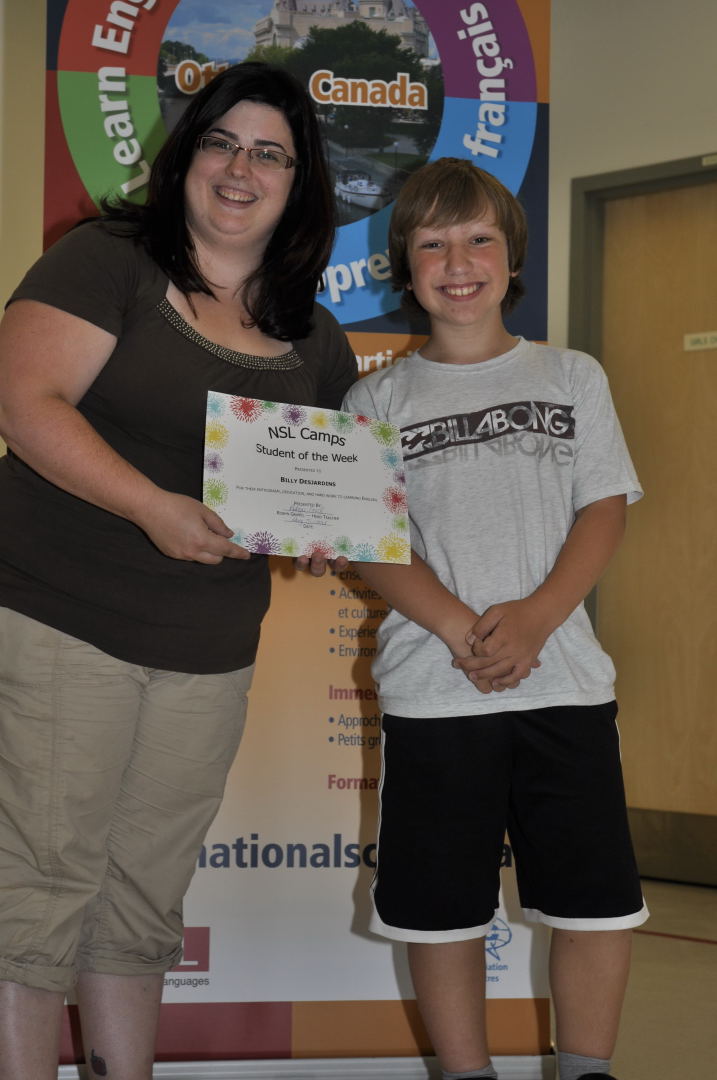In the image, a smiling teacher stands to the left of a young student. The teacher, appearing to be around 40 years old with black straight long hair and glasses, is holding up a certificate that reads "NSL Camps Student of the Week." She is dressed in a maroon, short-sleeve blouse with decorative detail at the collar, and tan pants that go up to her knees. The student, approximately 10 or 11 years old with long, dirty blonde, surfer-style hair, wears a gray Billabong t-shirt with a black rectangular background and black shorts with white stripes on the sides and bottom. His hands are crossed at his waist. Behind them, there is a circular advertisement banner featuring the words "Learn English, Français" and something about Canada, possibly "Ottawa." A wooden classroom-style door is visible in the background.